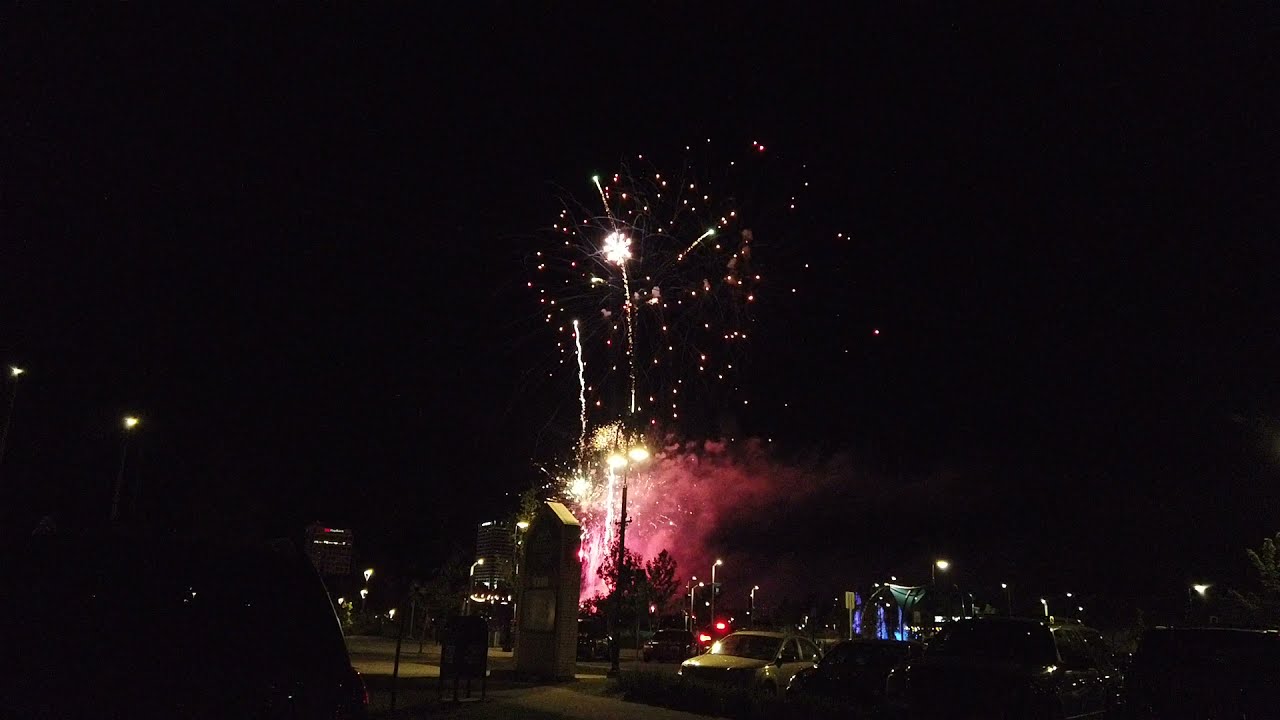The image captures a vibrant nighttime fireworks display, with around four fireworks bursting in unison across the sky. The fireworks showcase bright white and yellow explosions, accompanied by vivid yellow hues and trailing pink smoke. The scene is set above a sprawling parking lot, reminiscent of those found at sports stadiums, filled with parked vehicles. Surrounding the parking lot is a townscape featuring mid-rise buildings, approximately 12 stories high. The foreground is dominated by the parking lot, which contains some street lamps and various structures. Among them is a kiosk-like structure with a slanted roofline, a trash can nearby, and a stone structure with a sign. In the distant background, a blue-illuminated fountain adds a subtle glow to the darkened surroundings. The overall ambiance is characterized by the contrast between the bright fireworks and the dark night, with no visible people, accentuating the nocturnal festive spectacle.